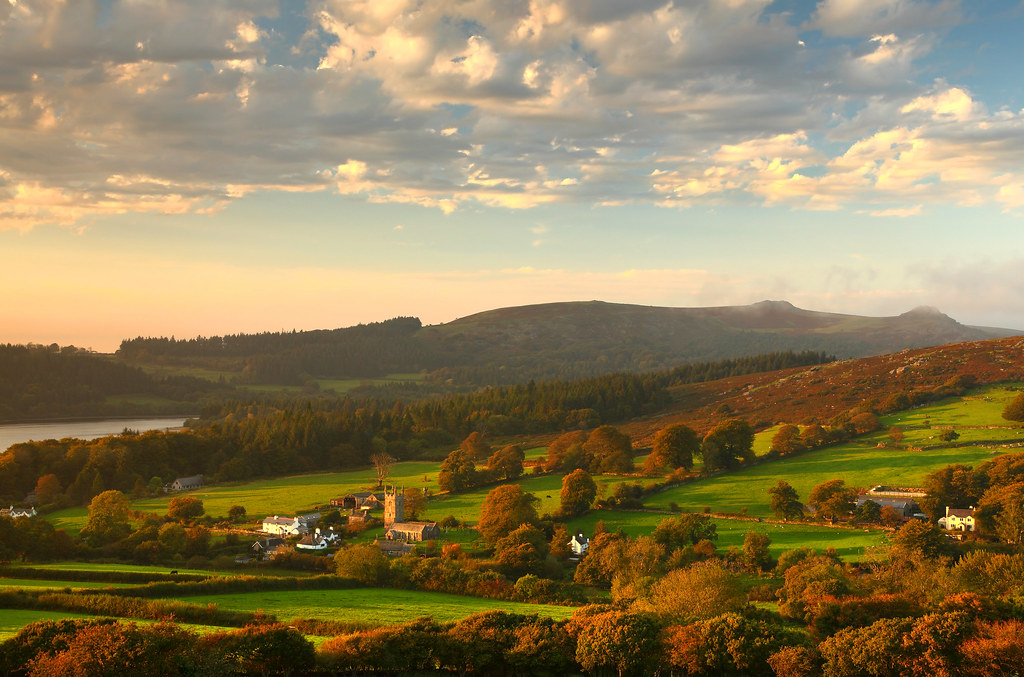A picturesque scene featuring a vibrant blue sky adorned with fluffy, white clouds. The landscape below showcases lush green trees interspersed with striking crimson-red foliage, indicating the beauty of the transitional season. Expanses of verdant grass spread across the foreground, leading to an assortment of charming buildings in the background. The architectural styles and general ambiance suggest a quaint town, possibly located in Europe.